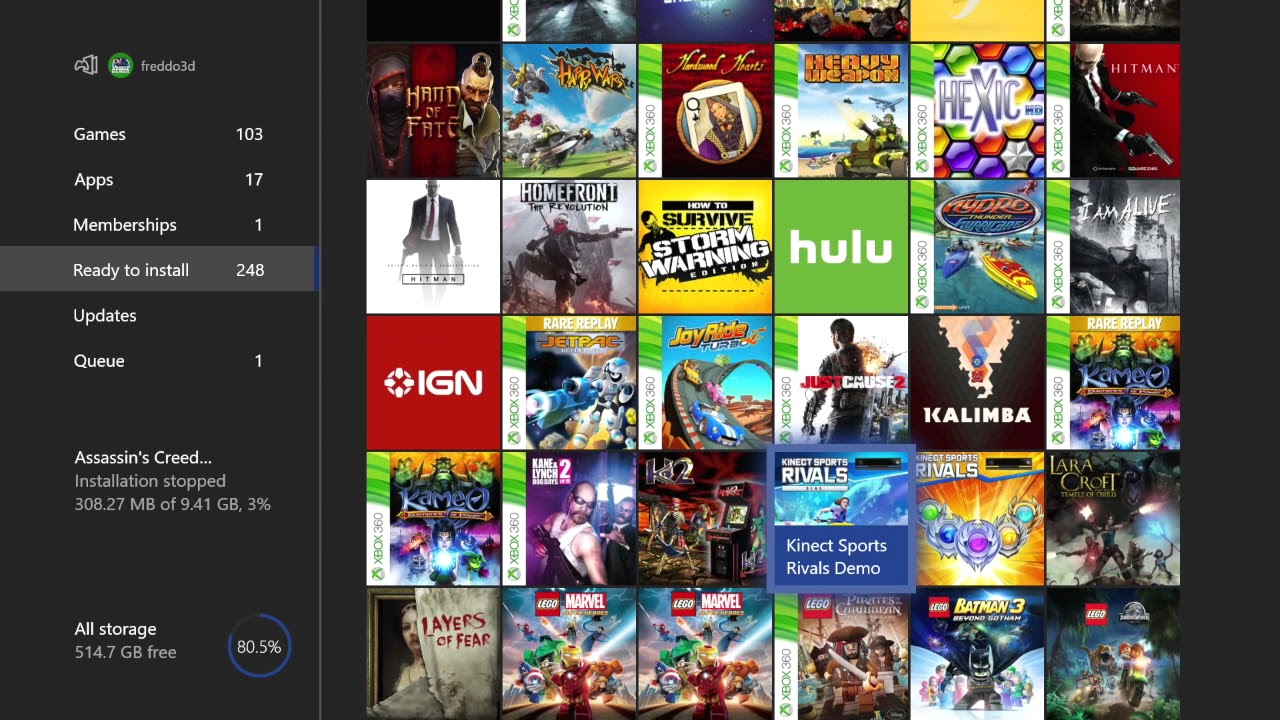The screenshot captures the Xbox interface, specifically the section where users can manage their games and applications. The interface displays various menu options including "Games," "Apps," "Memberships," "Ready to Install," "Updates," and "Queue." Below these menu options, there is a notification indicating that the installation of "Assassin's Creed" has stopped, with a progress status of 308.27 megabytes. The total storage available is listed as 514.7 megabytes. The screen also shows a list of games and applications, which includes "Hand of Fate," "Heavy Weapon," "Hexic HD," "Hitman," "Hulu," "Homefront," and "IGN."